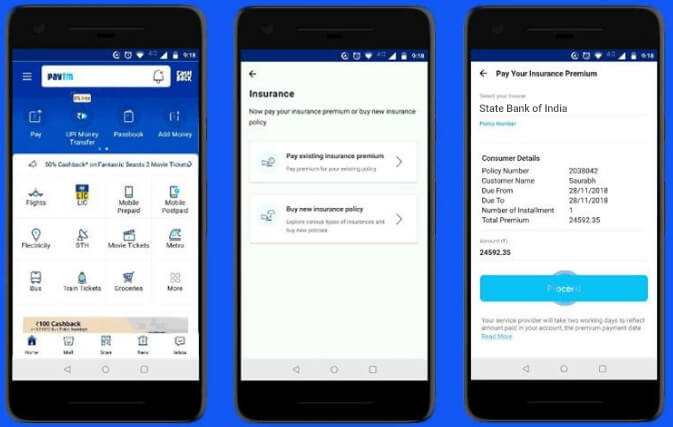In the image, three identical cell phones are displayed side by side against a bright blue background. Each phone features a black bezel that is thick on the top and bottom but thin on the sides, with rounded corners and a gray outline encircling the devices. 

The screen on the first phone shows a user interface with a large blue header containing a white search bar on the left, which has a blue, blurry logo that's indistinguishable. To the right of this search bar, the words "CASH BACK" appear in white text, with "CASH" positioned above "BACK" in a slightly curved or arching manner. Below this header, four options are displayed against the blue background: 

1. "PLAY" enclosed in a thin white outline with a white blob in the top right corner.
2. A second option with blurred, unreadable text and another white blob.
3. An icon of a white clipboard labeled "PASSBOOK."
4. Another icon with illegible white text beneath it, labeled "ADD MONEY."

Further down the screen, a section with a white background shows multiple icons representing different services. From left to right, the icons are labeled: "FLIGHTS," "LIC," "MOBILE PREPAID," "MOBILE POSTPAID," followed by another row with: "ELECTRICITY," "STH," "MOVIE TICKETS," "METRO," "BUS," "TRAM TICKETS," "GROCERIES," and "MORE."

The screens on the other two phones display various pieces of financial information but are less detailed in terms of specific content visible in the image.